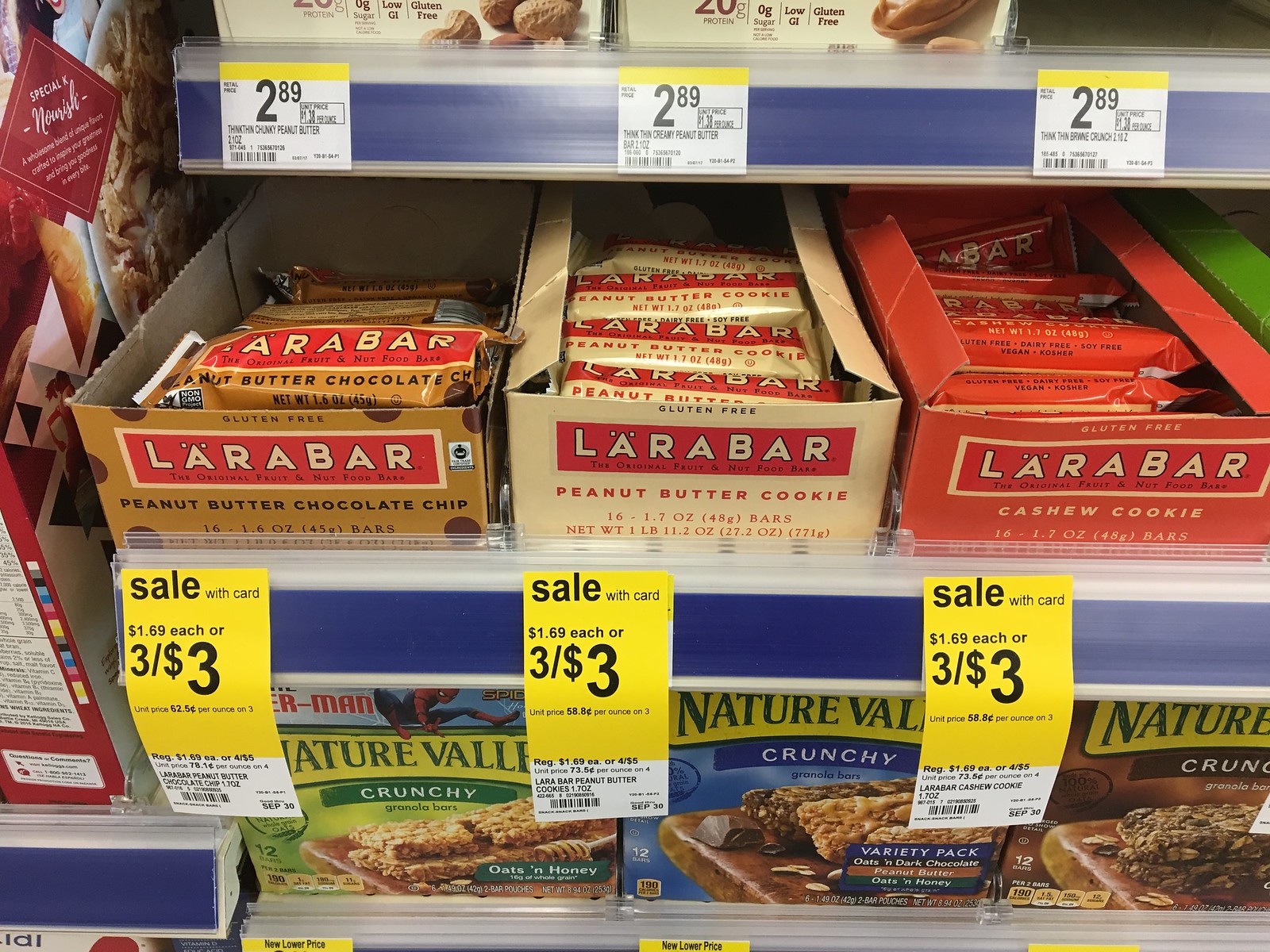This photograph captures a zoomed-in view of a store display featuring two popular brands of granola bars, predominately occupying the middle shelf. Central to the image are three varieties of Larabar granola bars, each distinguished by their distinct packaging: on the left is peanut butter chocolate chip in a light brown box with a red rectangle and beige block letters spelling 'Larabar'; in the middle is peanut butter cookie in a taupe, light beige box; and on the right is cashew cookie in a red-orange box. Below these, the display features three varieties of Nature Valley Crunch granola bars: oats and honey in a green package on the left, a variety pack in the middle, and a partially cut-off brown box on the right, likely dark chocolate flavored. Prominent sales tags are visible: a yellow sticker under the Larabars indicates they are on sale for $1.69 each or three for $3 with a card, and another label above indicates a $2.89 price point for another product. Adjacent to the Larabars are other nut-based and gluten-free products, contributing to a diverse and appealing snack display.